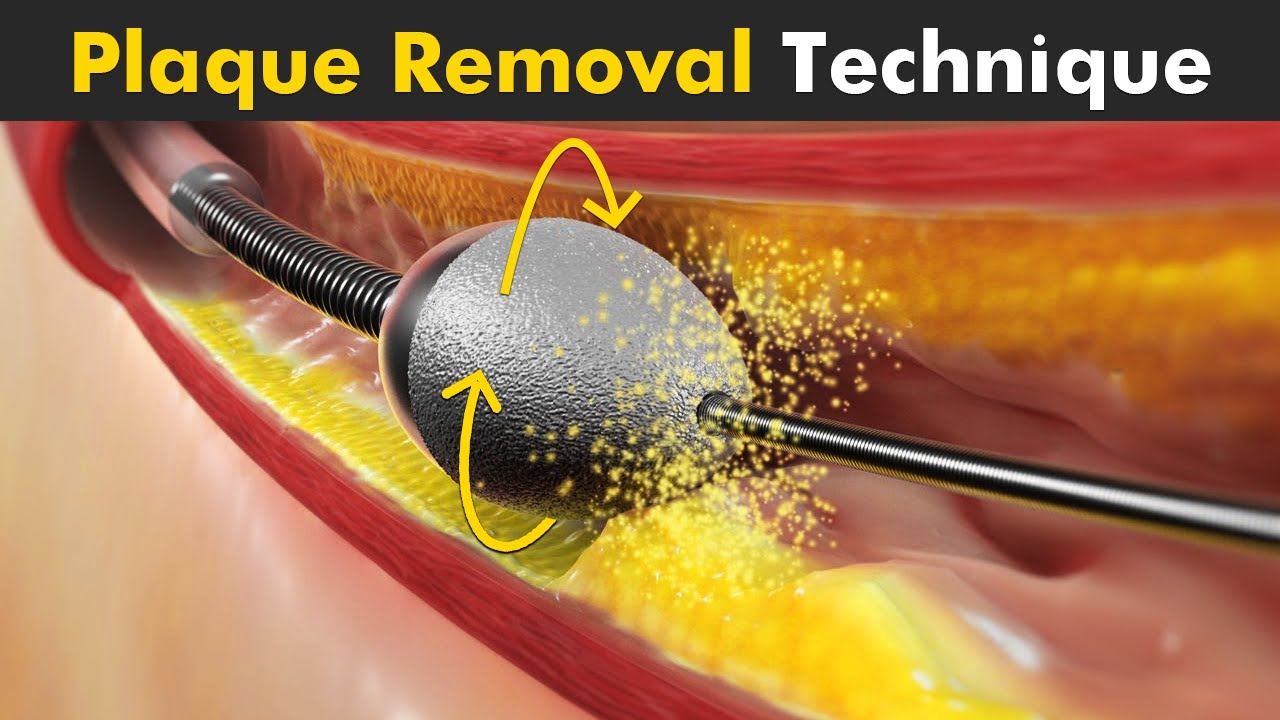The image appears to be an illustration from a medical publication, possibly an advertisement or poster typically found in a doctor's or dentist's office. The top of the image features a black bar with the text "Plaque Removal Technique"; "Plaque Removal" is written in yellow, while "Technique" is in white. Below the text, there is a detailed depiction of the inside of an artery or blood vessel, invaded by plaque highlighted in yellow. A sophisticated plaque removal device is shown inserted into the cutout artery. The device resembles a metal tubular tool with rivet-like features and a handle equipped with a spring for flexibility. Central to the illustration is an egg-shaped, rotating, spherical component of the device, encircled by two yellow lines with arrows indicating its rotational direction. This component appears to grind away the plaque, as indicated by auxiliary graphics showing the mechanism's action.